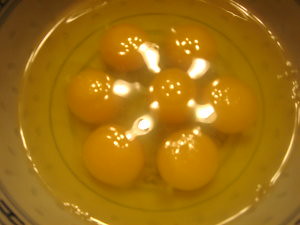A low-resolution, slightly out-of-focus colour photograph depicts a bowl containing seven whole egg yolks immersed in their whites. The bowl appears quite wide and features a decorative design, including what seems to be a green concentric ring circling below the surface of the egg whites. Due to the poor quality of the image, the exact colours are hard to determine. The lighting creates severe reflections and white hotspots predominantly in the central area over the egg yolks and intermittently around the meeting edge of the egg whites and the bowl, which may be ceramic with a white and blue or brown tint. The egg yolks themselves are notably vivid in yellow and orange shades, contrasting against the slightly yellow-tinted egg whites.